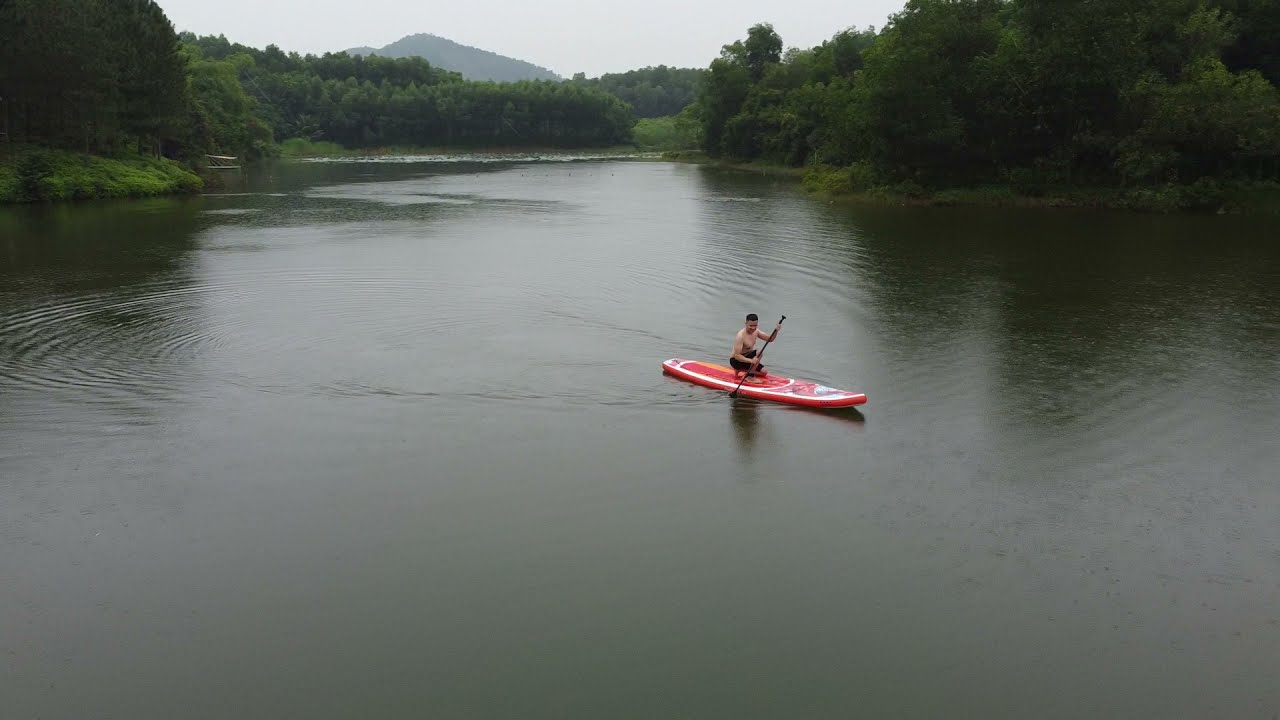In this serene and peaceful scene, a topless man with dark hair, wearing black shorts, is kayaking solo on a red and white kayak in a vast, somewhat overcast lake. The expansive lake, which takes up about three-fourths of the image, features murky green water with lighter patches where light reflects. Ripples spread outward from the kayak, creating concentric circles that disturb the otherwise calm surface. In the background, a dense forest of green pine trees and grass surrounds the lake, with the silhouette of distant mountains and hillsides adding depth to the landscape. The sky above is a narrow, grayish-white strip, hinting at the cloudy weather. The man, positioned in the middle right-hand side of the image, paddles steadily, adding to the overall tranquility of the scene.